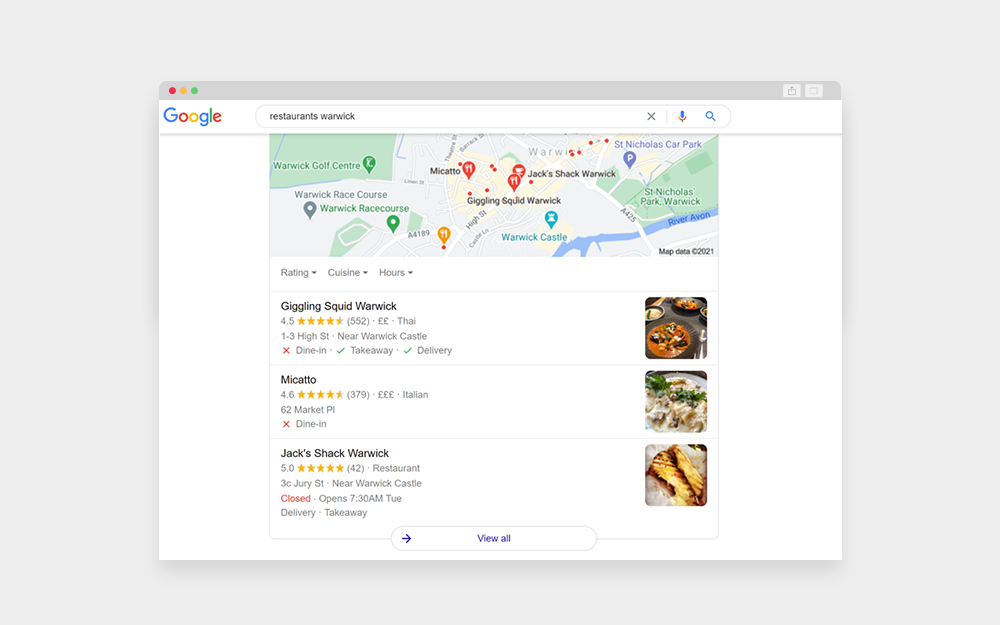This image is a screenshot captured from a Mac, as evident by the red, yellow, and green window control buttons located at the top-left corner. The screenshot displays a Google search results page for "restaurants Warwick." The search results prominently include a map with three restaurant locations marked.

1. **Giggling Squid Warwick**:
   - **Type**: Thai Restaurant
   - **Price Range**: ££ (Moderate, approximately $20 per plate)
   - **Rating**: 4.5 stars from 552 reviews

2. **Mikado**:
   - **Type**: Italian Restaurant
   - **Price Range**: £££ (Expensive, indicating a more upscale dining experience)
   - **Rating**: 4.6 stars from 379 reviews

3. **Jack Shack Warwick**:
   - **Rating**: 5 stars from 42 reviews

The layout centers around these top results, providing both brief descriptions and ratings, and situating them on the accompanying map for easy reference.